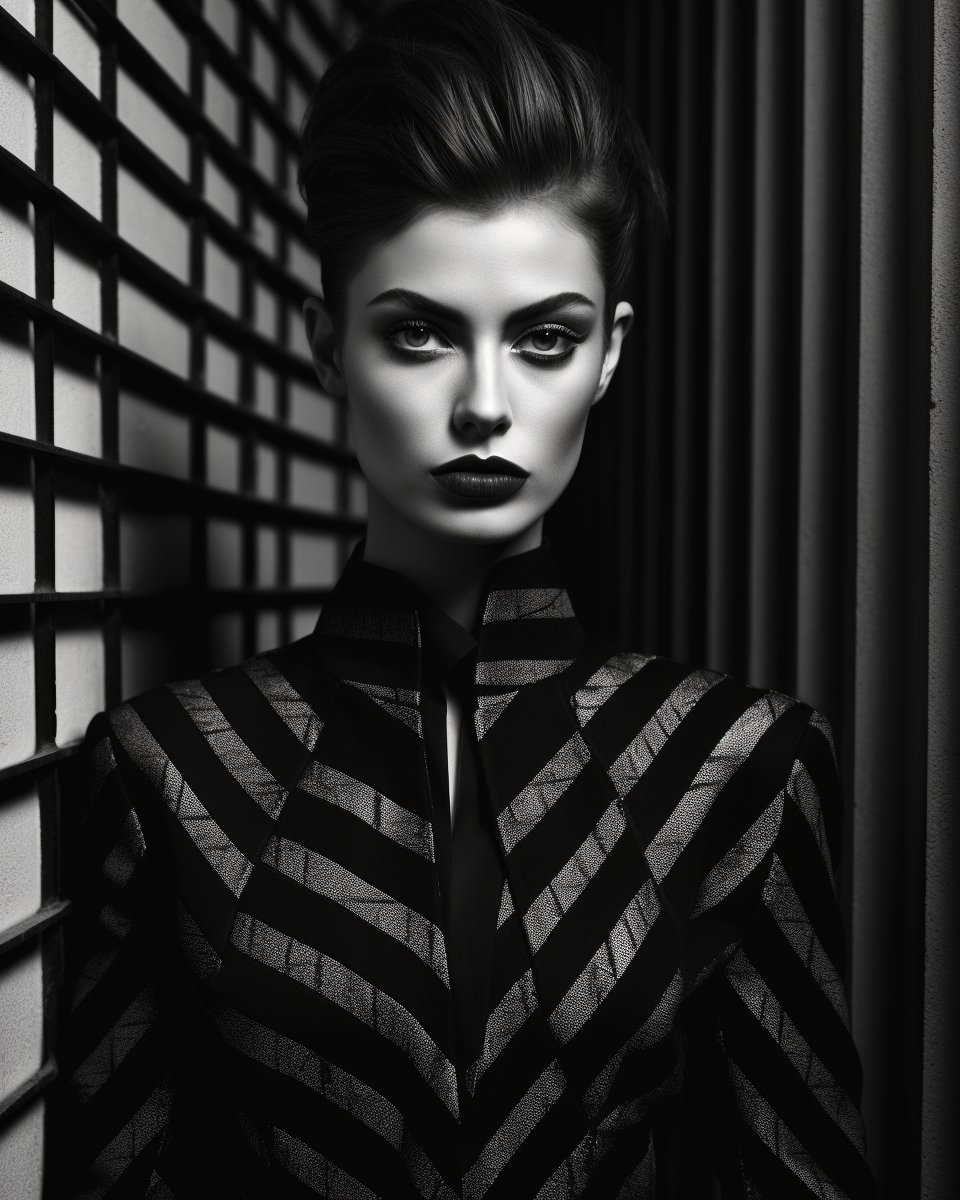This captivating black and white photograph features a young female model standing in a tightly spaced corridor, exuding an evocative blend of modern and retro styles. The composition is meticulously crafted with an emphasis on geometric shapes and contrasting textures. The model, adorned in a distinctive blouse composed of black and silver strap material, is accented by a grid-patterned wall on her left, resembling a Japanese screen made of dark wood against a lighter background. On her right, a dark curtain frames her figure, enhancing the visual drama.

Her striking appearance includes slicked-back dark hair, meticulously applied makeup with dark eyebrows, and bold red lipstick, producing a look reminiscent of the Bride of Frankenstein. Her expression is subtly amused, adding depth to the composition. The interplay of lighting accentuates her face and the textures around her, while her blouse features diagonal stripes with intricate designs, contrasting against the vertical lines of the corridor's right wall and the crosshatched grid pattern on the left. This photograph masterfully captures a blend of dark shapes, colors, and geometric elegance.